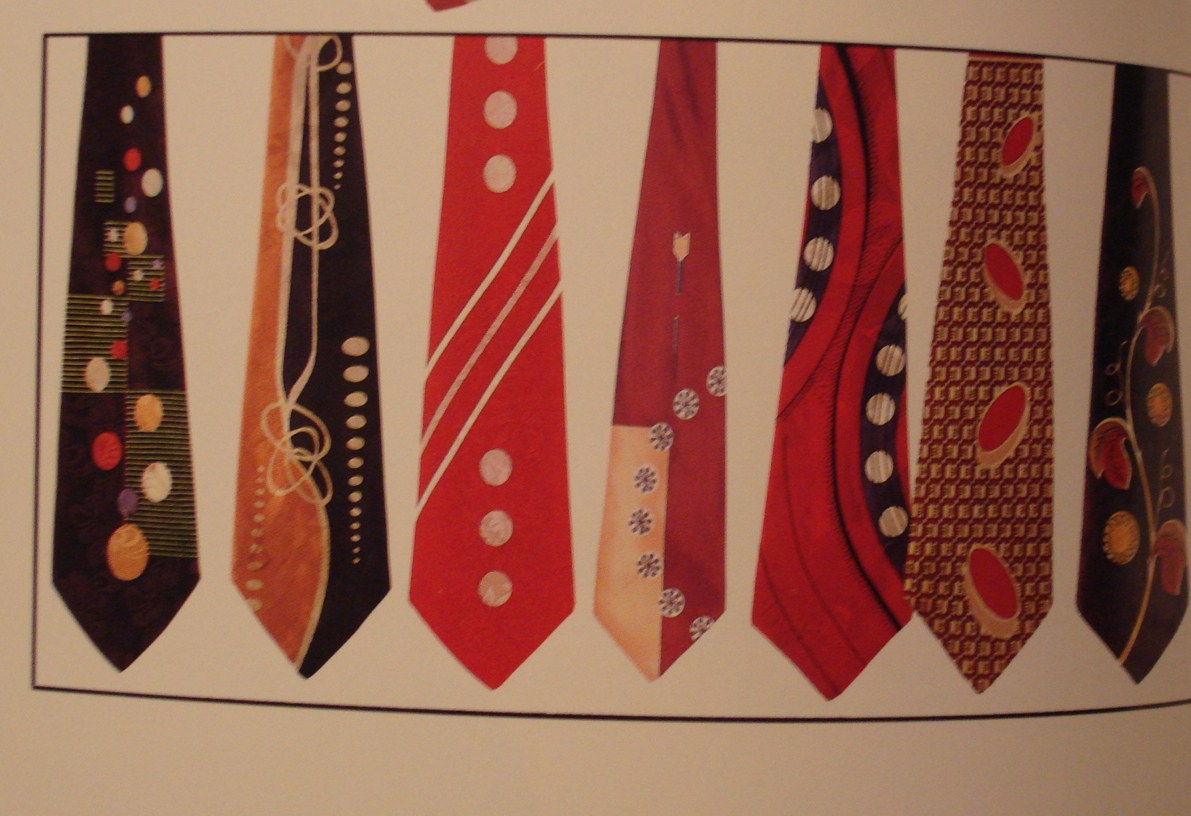The image is a blurry, poorly lit snapshot of a page from a book or catalog, depicting an artistic arrangement of seven neckties with bold, vibrant designs, reminiscent of the 80s or early 90s. These ties, illustrated in various colors such as blue, red, white, orange, black, purple, yellow, and brown, feature complex patterns including squiggles, spots, flowers, circles, and planetary motifs. Each tie showcases a unique combination of colors and designs: one with square pieces of yellow lines on a black and brown background, another with planets of different colors, a tie divided into orange and black sections by a white twirling ribbon, one maroon tie with white circle patterns, another red tie with peach shield-like symbols flanked by snowflakes, a red tie with curved black swatches containing white circles, and a brown tie adorned with circular pieces in red and beige. The page appears slightly bent, adding to the impression of a physical book or catalog page. The entire image carries a tungsten lighting ambience, contributing a yellowish hue to the photo.